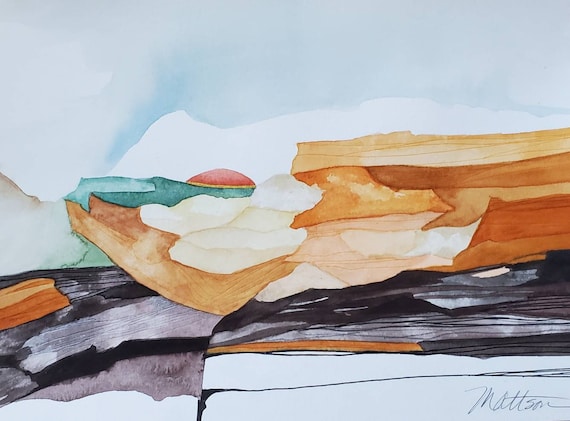The image depicts a rectangular, approximately four-inch wide by three-inch high watercolor painting of a serene sunset scene. At the top, a soft light blue sky transitions into deeper periwinkle hues, capturing the essence of dusk. Silhouetted against this sky is the striking red top quarter of the setting sun, casting a mellow glow. Below the sun, the tranquil ocean is painted in soothing aquamarine tones. The right side showcases layers of earthy tones—light brown, tan, reddish brown, and cream—that evoke the texture of eroded cliffs or rugged mountainsides. Interspersed throughout are darker veins of black, steel gray, and lavender, adding depth and contrast. Additionally, a notable dark green patch beneath the sun adds a touch of mysterious vibrancy. At the lower right-hand corner, the artist has delicately signed their name, "Mattson," in pencil or pen, finalizing the piece with a personal touch.